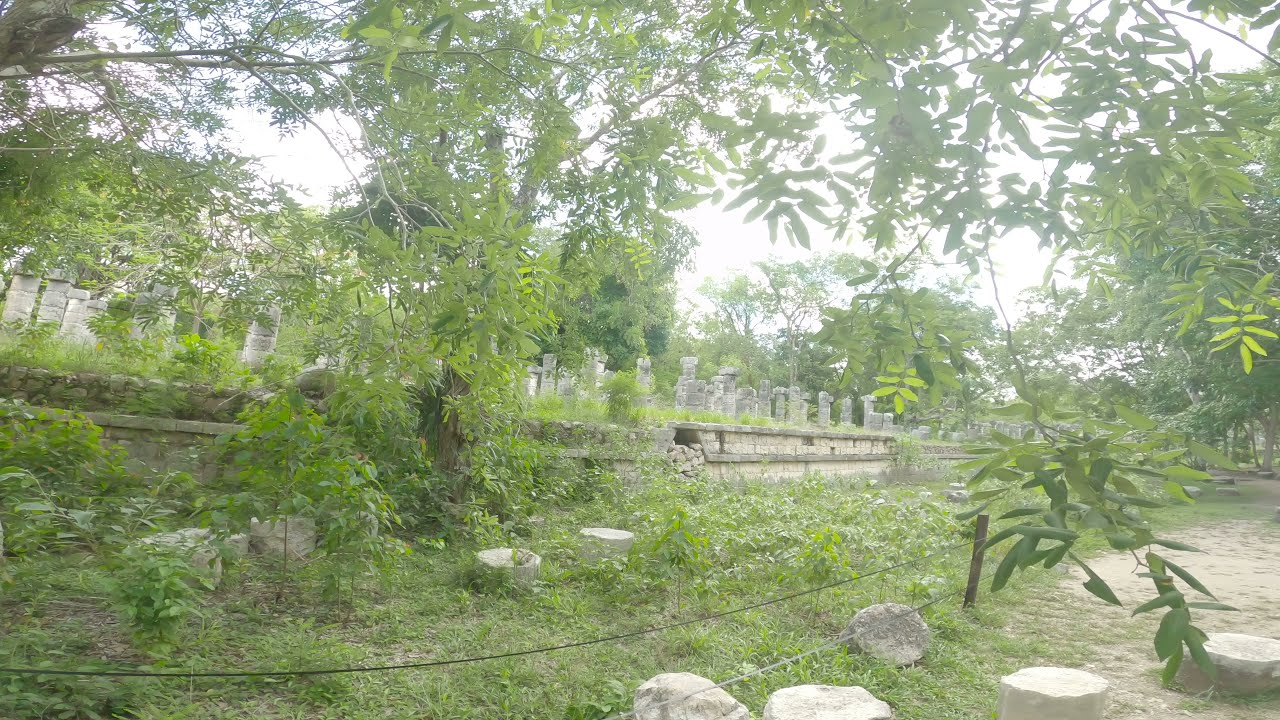This horizontally aligned rectangular image captures the edge of a cemetery or possibly an ancient ruin site during daylight hours. The scene is lush with greenery, featuring numerous trees with low-hanging, vibrant green leaves and clusters of thin leaves grouped in fives. The sky above is bright, almost white, casting an off-colored light over the area. 

In the background, the slightly elevated area is populated with an array of standing gray stones, hinting at either gravestones or ancient stone pillars, meticulously organized. These stones are bordered by a retaining wall which separates them from the lower grassy ground level where the photo is taken. 

In the foreground, at ground level, there are scattered large rocks, circular stones, and a gravel pathway visible in the bottom right corner. This lower area is partitioned from the raised section by a fence made up of either wooden or metal posts and wire. The photo has a somewhat blurry quality, adding to the mysterious ambiance of the place. There are no people or text visible in this predominantly green and serene landscape.